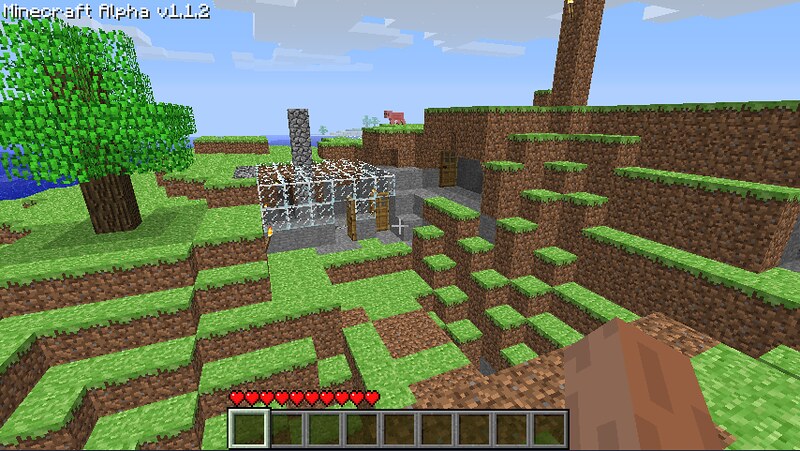A nostalgic screenshot captures an individual playing an early version of Minecraft, specifically Alpha v1.1.2. In this image, the player is in survival mode, having established a cozy base adorned with torches to ward off mobs. The primitive base, likely positioned near a few mines, features standard wooden doors – a visual reminder of the era predating the introduction of various door types. The presence of torches around the base highlights their crucial role in early gameplay for preventing mob spawns. Notably, the player has added a charming touch with a makeshift chimney extending from their glass house, evoking a sense of creativity and nostalgia. This screenshot serves as a wonderful throwback for long-time Minecraft enthusiasts, reminding them of the simpler times in the game's evolution.